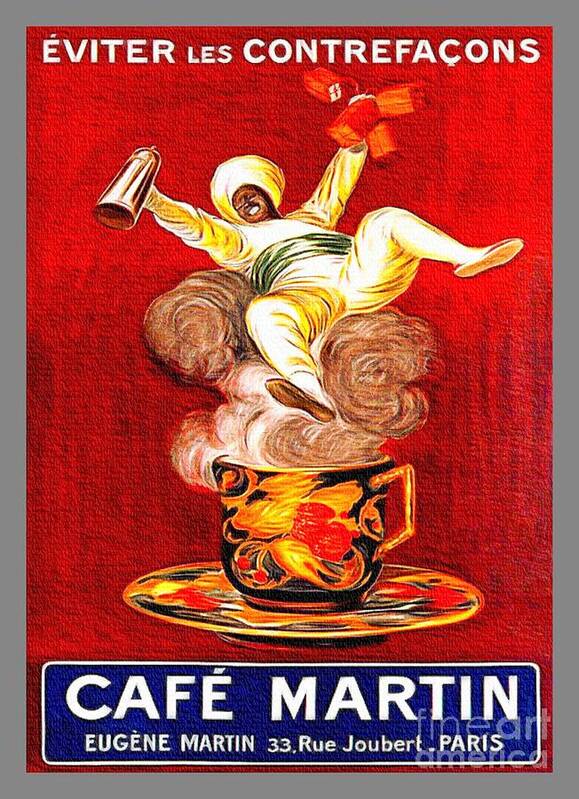This antique-style poster for Café Martine, located at 33 Rue Joubert, Paris, features a vibrant and whimsical design. Set against a predominantly white background with a painted style, the central image shows a cheerful chef dressed in white attire who appears to be riding a plume of steam emanating from an elegant black coffee cup adorned with gold floral embellishments. The chef, depicted holding a coffee carafe and possibly some sweets, sits atop this steam that rises from the cup, which rests upon a plate. Above this charming scene is the French text "Éviter les contrefaçons," and at the bottom, inside a blue rectangle outlined in white, is the café's information: "Café Martine, Eugène Martine, 33 Rue Jaubert, Paris." The poster's artistic details and playful imagery effectively communicate the warmth and allure of the café.